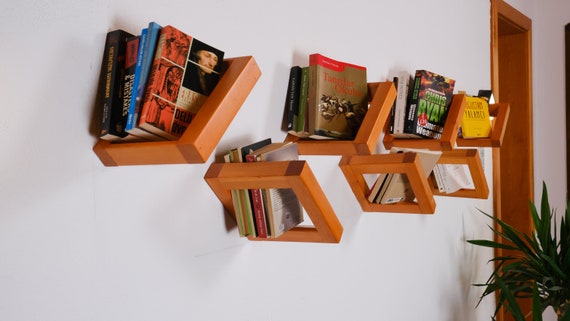In the image, a minimalist bookshelf composed of seven open square frames is mounted on a white wall. These squares are staggered and each tilted slightly in various directions, creating a dynamic visual arrangement. 

In the first square, which tilts gently to the right, there are five books. The second square, positioned behind the first, holds three books. The third square also contains three books. In the fourth square, the number of books isn't fully visible; however, one book stands out with its yellow cover adorned with black text. 

Below these, the fifth square is tilted backward and houses two white books. The sixth square, set behind, features three beige-colored books. Lastly, in the seventh square, there are about five books, with their spines in view, showing distinct colors: white, red, and green.

On the bottom right-hand corner of the image, part of a lush green plant is visible, adding a touch of nature to the scene. Adjacent to the bookshelf, a wooden doorframe subtly enters the frame on the left side, contributing a warm, rustic element to the overall composition.